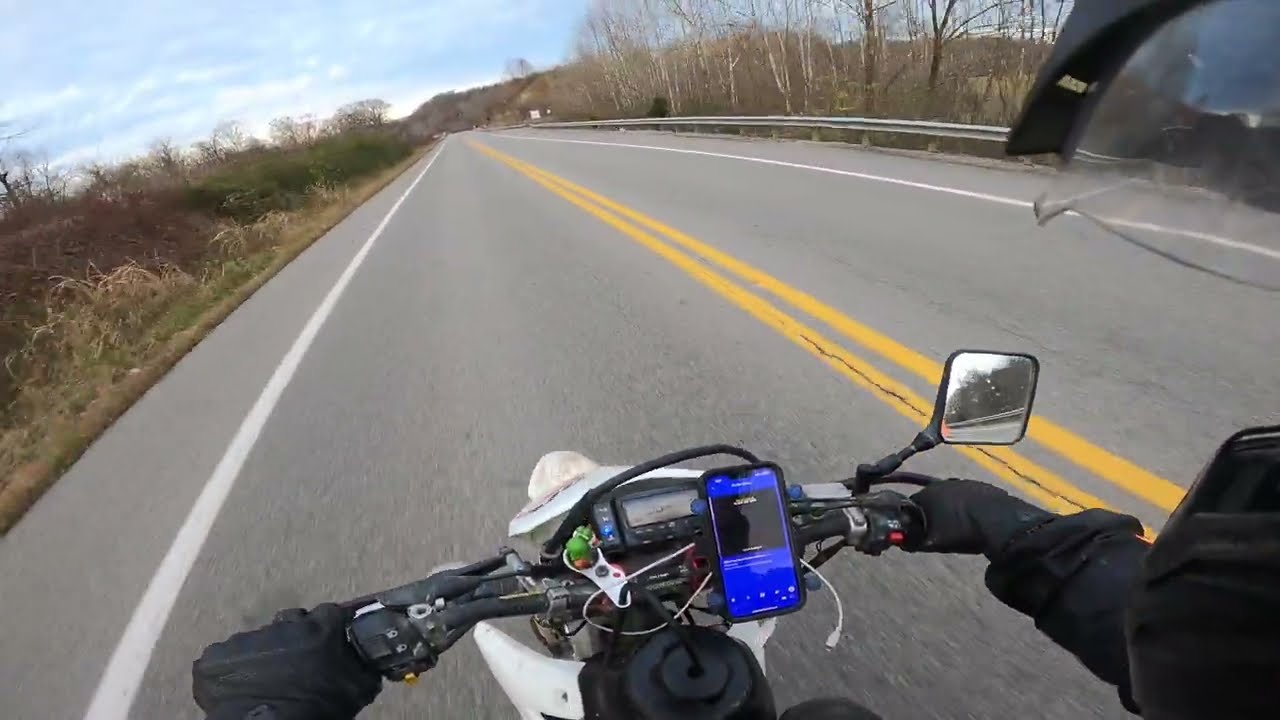The image is a wide rectangular photo showing a scenic two-lane highway lined with barren trees and partially green, brown brush. The road is composed of gray asphalt with white lines on the sides and a double yellow line running down the center. The road inclines slightly downhill on the left and features a silver guardrail on the right. The image is taken on a clear day with a blue sky and scattered white clouds.

In the lower section of the image, the front end of a motorcycle or scooter dominates the view. The vehicle has white bodywork and black handlebars. Attached to the handlebars is a smartphone with a blue screen, possibly used for navigation. The rider is visible from the waist down, wearing a black jacket and black gloves. Only their right arm and hand are distinctly seen gripping the handlebars, while a rearview mirror protrudes above the right hand.

The motorcycle is positioned in the left lane of the highway, which stretches forward and gradually narrows, disappearing into a distant brown hilly area topped by the sky. The rider’s direct view is framed by the handlebars and their right arm, with the double yellow lines leading the eye down the center of the image toward the horizon.